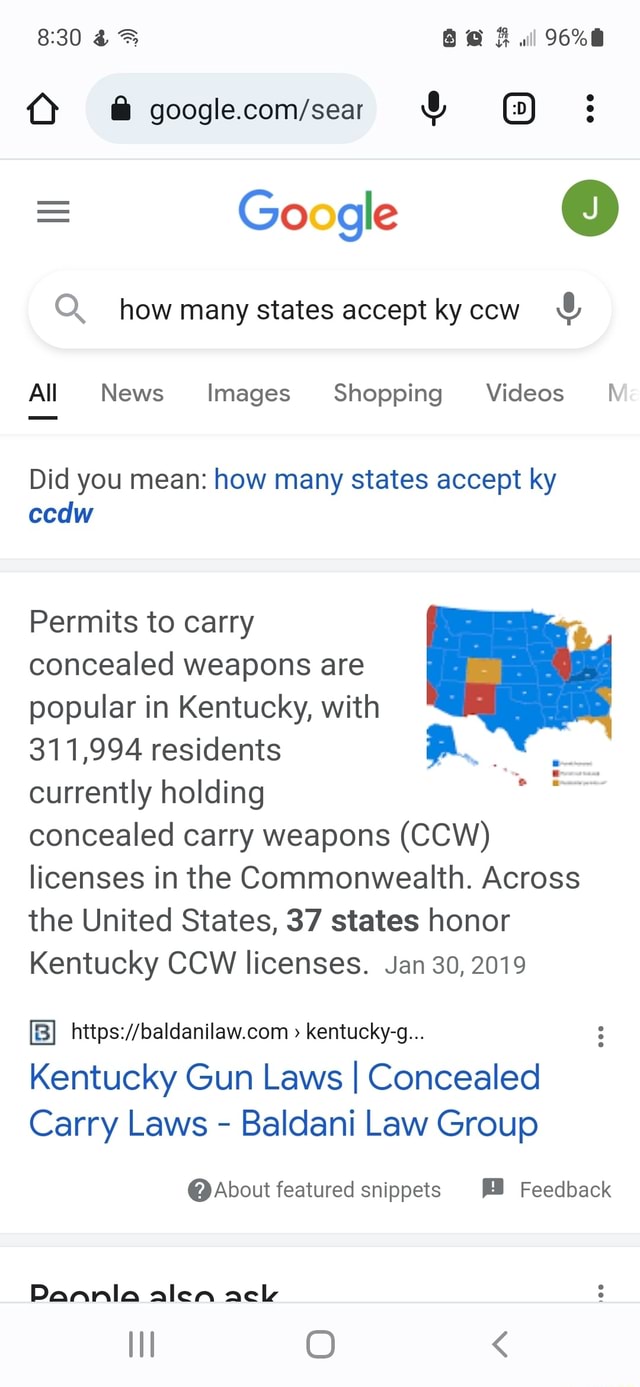The image depicts a Google search results page. At the top of the page, within the search box, there is a lock icon next to "google.com/search." The query typed into the search box reads, "how many states except KYCCW." Below the search box, the options for filtering results are listed as "All," "News," "Images," "Shopping," and "Videos," with "All" highlighted and underlined. There is a suggested correction for the query: "Did you mean how many states except KYCCW?"

To the right of this, there is a color-coded map displaying various states in blue, yellow, and red. To the left of the map, a snippet highlights the following information: "Permits to carry concealed weapons are popular in Kentucky, with 311,994 residents currently holding concealed carry weapon (CCW) licenses in the commonwealth. Across the United States, 37 states honor Kentucky CCW licenses." The information is sourced from a snippet dated January 30, 2019, attributed to balddannylaw.com with topics including "Kentucky," "Kentucky Gun Laws," "Concealed Carry Laws," and the "Baldanny Law Group." Below this snippet, there are links for additional actions like "About featured snippets" and "Feedback."